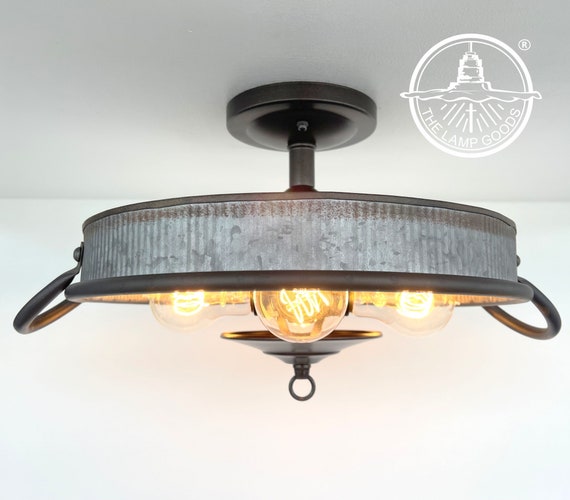The image features a distinctive ceiling light, designed to resemble an upcycled tin pan, commonly seen in contemporary bars and bistros. The light fixture comprises a round metal pan, appearing to be about two inches deep, with a rippled exterior and tubular handles on either side. Suspended from the center of the pan is a short, cone-shaped metal piece, blending seamlessly with the pan's material and coloring. Inside the pan are four visible filament-style bulbs, providing an artistic, old-fashioned aesthetic, though they are modern bulbs. The fixture is attached to the ceiling by a modern-looking mounting plate and rod. The background is a plain white ceiling and walls, indicating it is a product image. The top right corner features a logo for "The Lamp Goods," depicting an illustration of a lamp radiating rays, reminiscent of a lighthouse underwater with a cross.